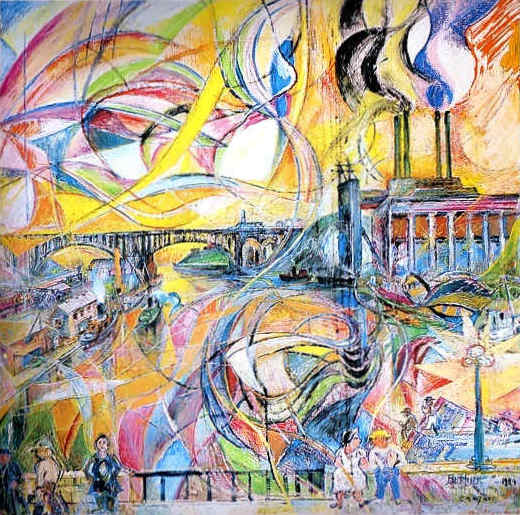This vibrant and eclectic painting is a captivating blend of abstract, cubist, and realistic styles, depicting a bustling city scene. The lower half of the painting features people walking and sitting along a bright, colorful boardwalk by a black railing, under a blue light post with globe lights. Some figures wear distinct attire, like a tuxedo with a bow tie. To the left, there's more activity with people scattered about, including a woman looking directly at the viewer. In the background, a large arch bridge spans across the scene, accompanied by a factory with prominent smokestacks emitting smoke. Further back is another bridge over water with docked boats and buildings featuring Roman-style pillars and windows. The sky and water are adorned with vivid, swirling, graffiti-like patterns in a myriad of colors—red, blue, yellow, green, purple—adding to the painting's dynamic energy. At the upper right corner, there's a mysterious face with blue eyes and a black smile, against a backdrop of swirling colors. This painting is a rich tapestry of shapes, lines, and hues, encapsulating a lively urban setting.